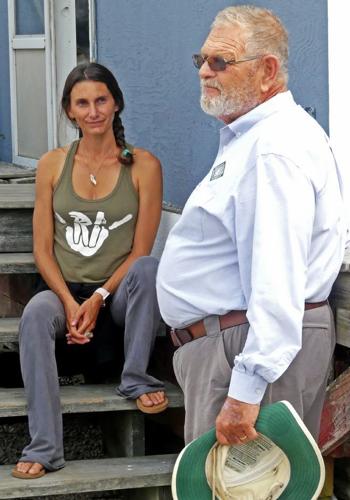In this photo, a woman with brown braided hair sits on the wooden steps of a slightly blue house, smiling subtly. She's dressed in a greenish tank top featuring a hand making the 'hang loose' gesture, light-colored sweatpants, and sandals. Seated on the second step from the top, her right leg rests on the bottom stair while her left leg is one step higher. Near her, a heavyset older man, possibly in his 60s with short gray hair and a neatly trimmed white beard, walks towards the steps while holding a cat. He's turned slightly away, carrying a cowboy hat with a green band in his left hand and wears sunglasses, a white button-up shirt, khakis, and a brown belt. The background shows a partially open door on the blue house.